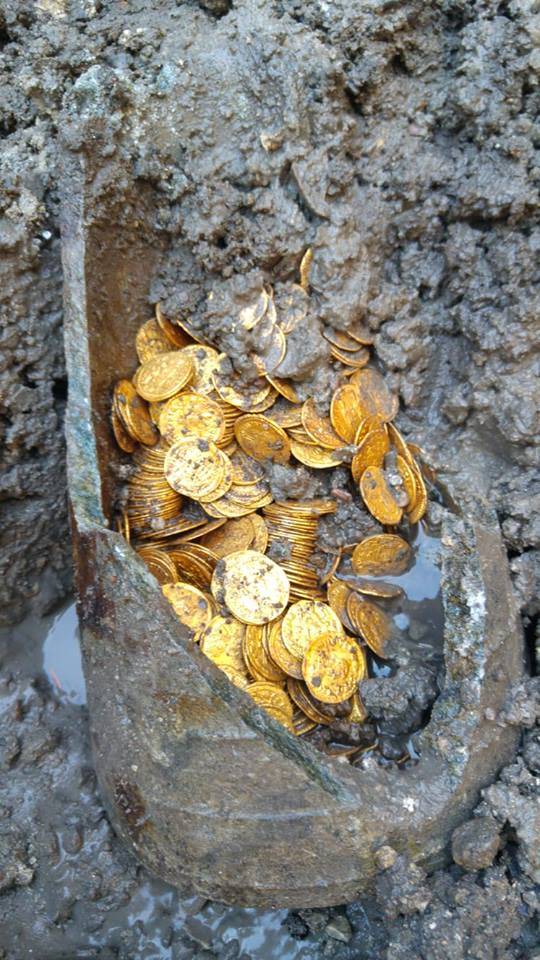The photograph captures an ancient, broken gray vessel, resembling a croc, partially unearthed in a muddy excavation site. This vessel, sitting on similarly gray stone, is still ensconced in soft dirt primarily along the top and right side, giving the impression of an ongoing dig. Dirt actively spills over and into the center of the croc, obscuring parts of it. The vessel's large, open front reveals a substantial hoard of glimmering gold coins or disks, although no markings or imagery confirm their exact nature. Water is pooled behind the croc in the back left corner, with additional small pools of water visible inside the damaged sections of the container, hinting at its recent removal from a likely water-rich environment. The croc and its contents are covered in mud, yet the gold coins still shine through, creating a striking contrast between the precious metal and the surrounding grunge. The background suggests continued digging activities, with hints of the excavation origin visible.